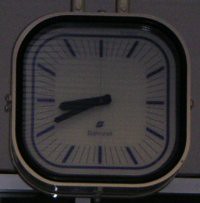This image depicts a compact clock with a minimalist design, suitable for a kitchen or as an alarm clock. The clock has a square shape with gently rounded corners at the top and bottom, giving it a sleek appearance. The casing seems to be made of molded plastic or possibly metal. A distinct black interior border frames the clock's face, which is light gray in color and also enclosed by a subtle, smaller border. The clock face lacks numerals, instead featuring simple markers to denote the hours. Traditional black hour and minute hands, along with a slender second hand, are mounted at the center. A small, indistinct logo hints at a brand name, although it is not clearly visible. The overall ambiance of the image is dim, casting shadows that add to its subdued character.